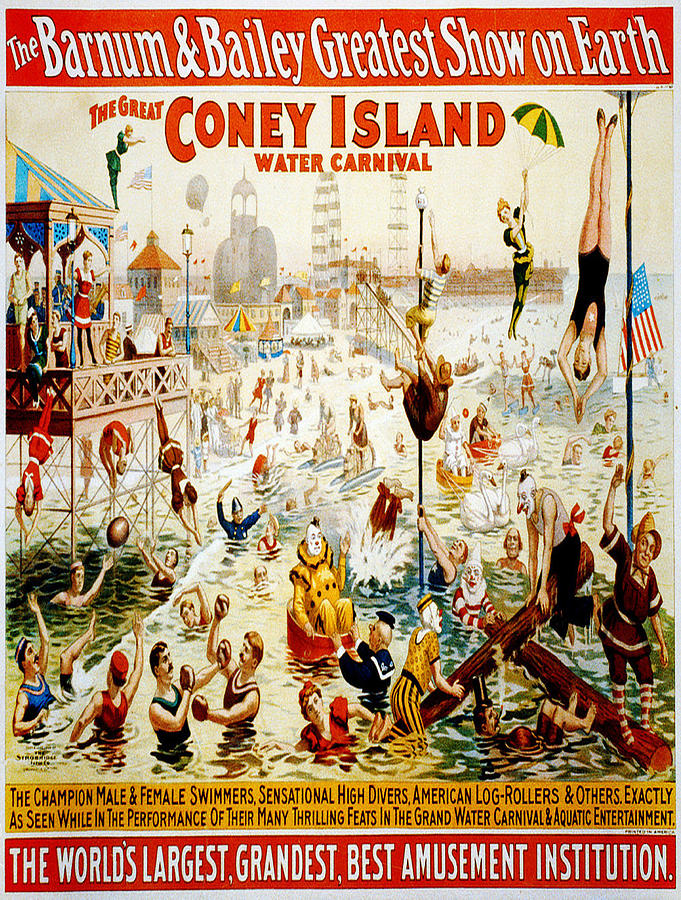This vintage poster for the **Barnum & Bailey Greatest Show on Earth** promotes the **Great Coney Island Water Carnival** in a vividly illustrated style. Splashed with an array of bright colors including red, white, yellow, blue, green, tan, black, and brown, the poster is a bustling scene of circus entertainment. The text at the top announces the event, reading "**The Barnum & Bailey Greatest Show on Earth**," while below in red letters it states, "**The Great Coney Island Water Carnival.**" 

The foreground features clowns and circus performers swimming and playing in the water. On the bottom left, two men are engaged in a boxing match, while nearby another group of men tosses a ball. A small building on stilts stands to the left, from which performers dive into the water. The vibrant background is filled with iconic circus elements like tents, an American flag, a hot air balloon, and ferris wheels. 

In the lower section of the poster, a gold-colored bar spans the width, displaying black text that reads: "**The Champion Male and Female Swimmers, Sensational High Divers, American Log Rollers, and others, exactly as seen while in the performance of their many thrilling feats in the Grand Water Carnival and Aquatic Entertainment.**" Below this, a red ribbon carries white text proclaiming, "**The World's Largest, Grandest, Best Amusement Institution.**"

The scene encapsulates the lively atmosphere of the circus, featuring not just swimmers and divers, but also log rollers, acrobats, jugglers, a police officer with a bat, and even a giant slide. This captivating poster serves as an advertisement for the spectacular circus carnival held at Coney Island.